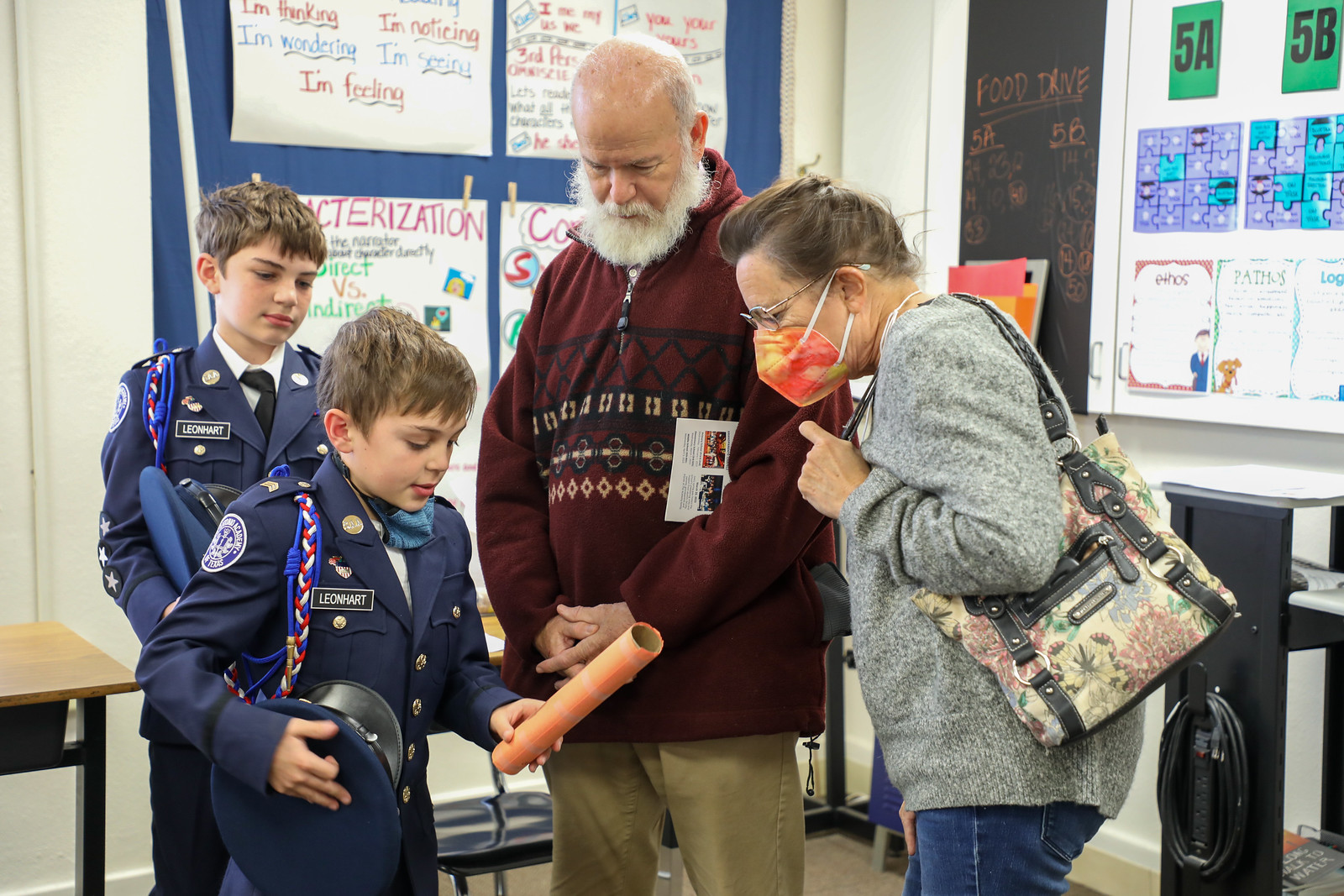This photograph captures a heartwarming moment in what appears to be a school classroom. The horizontal, rectangular image features two young boys, who seem to be around ten years old, dressed in formal blue uniforms reminiscent of a military school or scouting organization. They are clad in white shirts, blue jackets adorned with name tags, badges, and braids over their right shoulders. The younger boy, with slightly lighter hair, has a mask around his neck and is focused on showing a paper towel roll to the elderly couple beside him. The older boy, with dark brown hair, is also engrossed in the activity. Both boys hold blue hats in their hands.

Standing next to them are two elderly figures, likely their grandparents. The grandfather, wearing a maroon sweater and khakis, has a bald head and a bushy white beard. The grandmother, leaning in to get a closer look, is dressed in blue jeans, a gray sweater, and an orange face mask. She sports short, dark hair held back and carries a colorful purse. The background reveals a typical classroom setting with posters, children's schoolwork on the white walls, and the presence of desks and chairs, completing the scene of familial interaction and learning. All individuals appear to be Caucasian.